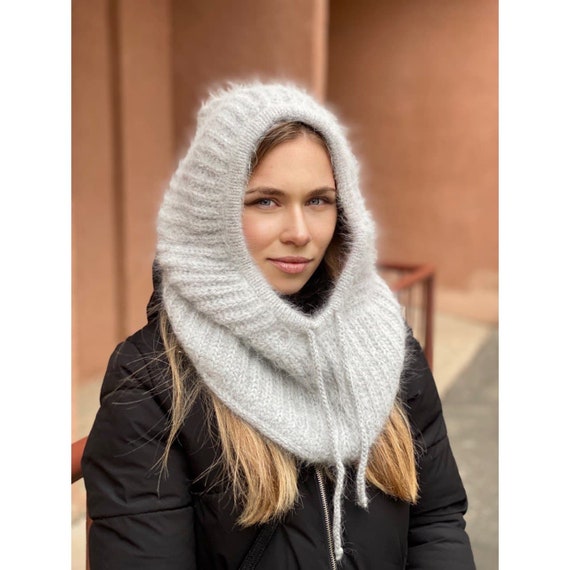The image features a young, blonde woman with a noticeable Russian appearance, captured in a well-focused photograph with a blurred background. She is dressed warmly in a black, poofy parka with the hood down, and her dirty blonde hair peeks out from beneath a distinctive and cozy knitted wool headpiece. This headpiece is light grey, almost white, and extends from the top of her head down to her chest, featuring long strings that hang down and could be used to adjust the fit around her face. The headpiece is fuzzy with little wool fibers, enhancing its winter charm. The woman is either standing or leaning near a stairwell or metal frame, and behind her, blurred brown walls can be seen. She gazes at the camera with a subtle smile, exuding a sense of warmth despite the wintery attire.